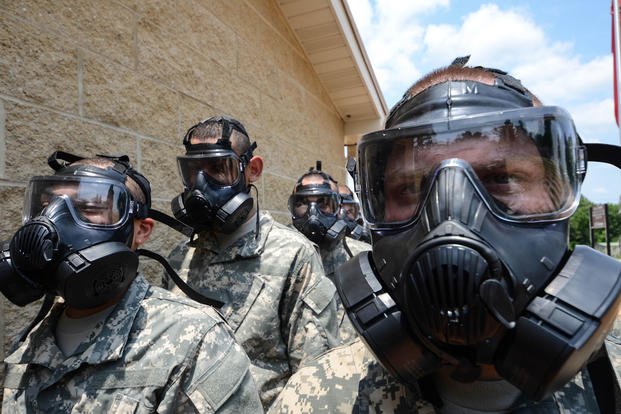In a horizontally aligned, rectangular close-up photograph, a group of military soldiers is depicted walking beside a light brown stone wall. Each soldier is clad in a camouflage uniform with beige and green hues, and they all wear thick, black gas masks equipped with integrated goggles. These gas masks appear to be made from a leather-like material and fully cover their faces. The soldiers, characterized by their shaved brown heads, are seen progressing in a formation that includes a front soldier and lines extending behind him, ultimately forming a double-file line.

The prominent figure in the foreground is captured from the right side, revealing just a part of his head and a glimpse of his camouflage uniform. To the left of him, the continuation of the line of soldiers can be seen, with each individual similarly equipped and attired.

In the background, the upper right corner of the photo reveals a clear blue sky interspersed with white, puffy clouds. Additionally, there are some distant trees and a wooden sign with white text, supported by two posts on the right edge of the image. This detailed scene conveys a clear sense of the soldiers' uniformity and readiness, as they march in their protective gear along the wall.